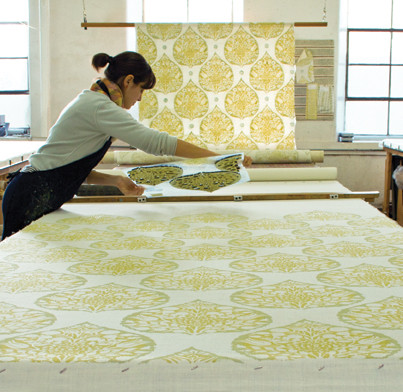The photograph captures a focused scene of a woman, potentially a designer or artisan, diligently at work in what appears to be a tapestry mill. Positioned on the left side of the image, she is dressed in a black apron over a white long-sleeve shirt, with the sleeves rolled up to her elbows, and an orange and yellow handkerchief around her neck. Her dark hair is pulled back into a ponytail, ensuring it stays out of her way as she works. 

The woman is in the process of creating a pattern on a large piece of fabric spread across an expansive, white rectangular table. With a sizable stencil—about a foot long—in her hand, she’s pressing it down onto the material to form a repeating pattern of an oval or spade-like shapes against a cream-colored background. The forefront of the image showcases numerous instances where she has already applied the stencil, revealing the methodical design process. Rolled-up portions of the fabric await her attention.

In the background, a wooden dowel suspended by wires from the ceiling holds additional fabric, which drapes down elegantly and curls at its end. White walls and three large windows form a serene, well-lit backdrop for this meticulous craftwork. Additionally, a wooden measuring stick rests on the table, hinting at the precision required in her work. The setting is clean and minimalistic, keeping the focus on the intricate artisan technique and the tactile beauty of the fabric and its emerging design.